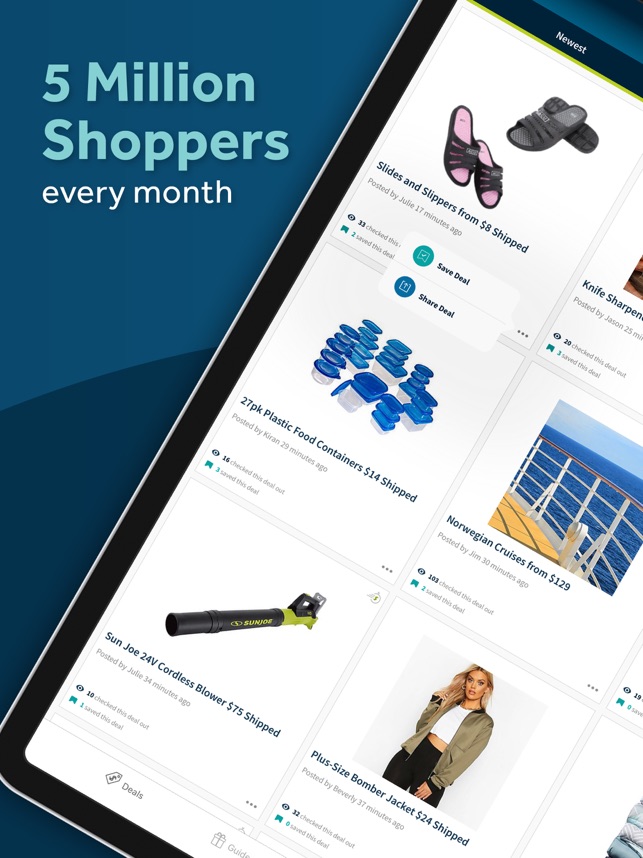The image depicts a tablet or iPad angled to the side against a teal background. The background features the phrase "Five million shoppers" in lighter teal text, with "every month" in white print below it. 

On the screen of the tablet, various shopping deals are displayed in square sections:

- In the upper-left corner, slightly tilted, the text reads "Slides and slippers from $8 shipped."
- Moving downwards, a partially visible label indicates a "Knife sharpener," although it is cut off.
- Further down, a deal for a "27-pack plastic food container for $14 shipped" is displayed.
- Following that is an offer for "Norwegian cruises from $129."
- On the lower part of the screen, there are more deals, such as a "Sun Joe 24V cordless blower for $75 shipped" and a "Plus-size bomber jacket for $24 shipped."
- The very bottom shows what appears to be a cut-off image of teal-colored sheets or similar items.

Some deals are only partially visible due to the angle and cropping of the image.